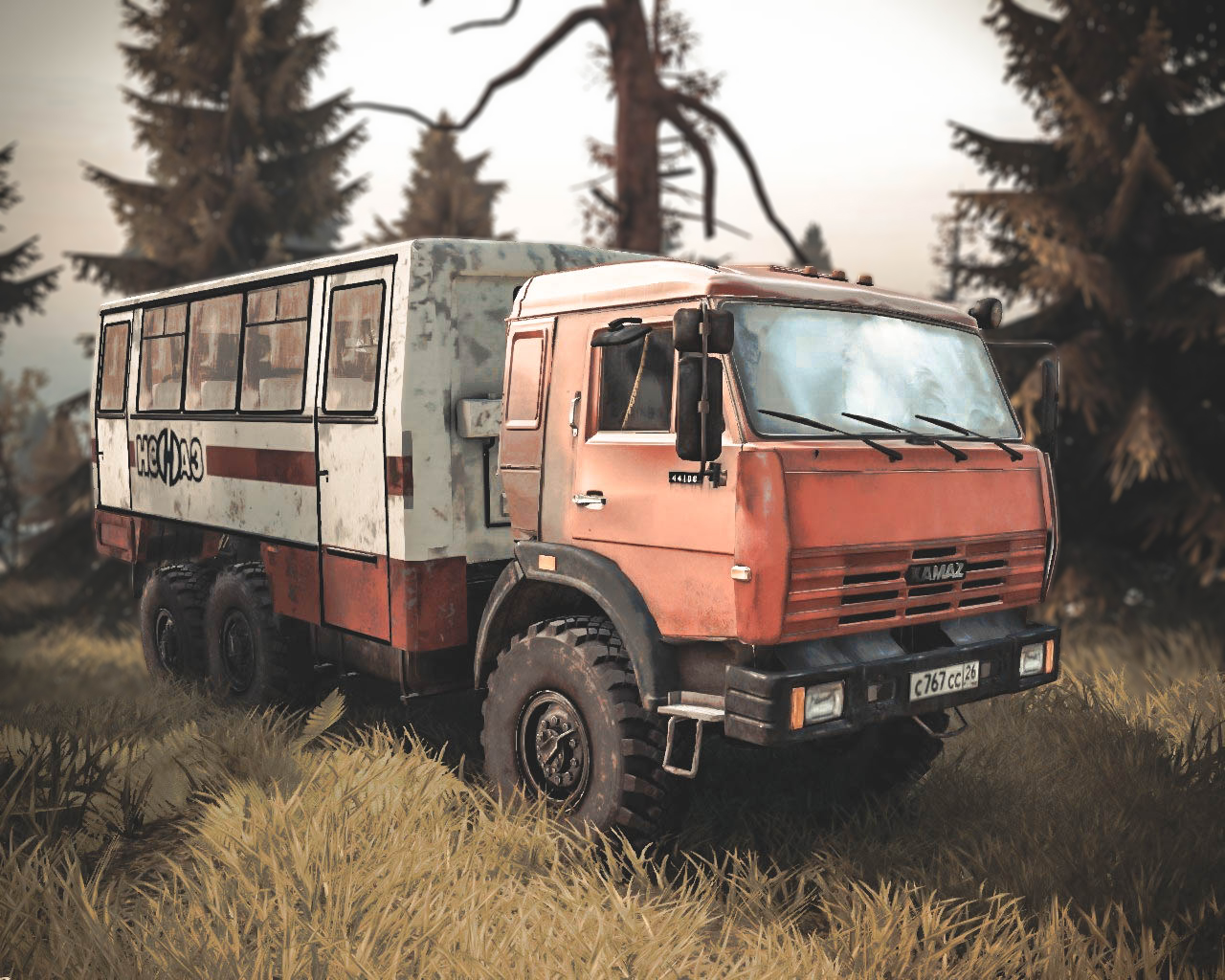A color photograph captures a Eurostyle minibus, identified by its K-A-M-A-Z branding on the front, parked in the middle of a field with mostly brown grass and a few green trees under a light gray sky. The minibus, which resembles a small semi-tractor trailer cab, appears to be decaying but doesn't seem to have been abandoned for very long. Positioned diagonally, the bus's engine area faces the bottom right, while its rear is to the left center. The front end is light red, and the sun-blocked windshield subtly conceals white seats inside, visible through large side windows outlined in black trim. The top portion of the bus's rear is white but dirty, transitioning to red at the bottom. The side features two thin doors with handles and windows, and the bus's license plate reads C-7-6-7-C-C-2-6. In the scenic background, a few birds fly near a tree with broken limbs, adding to the abandoned aura of the scene.